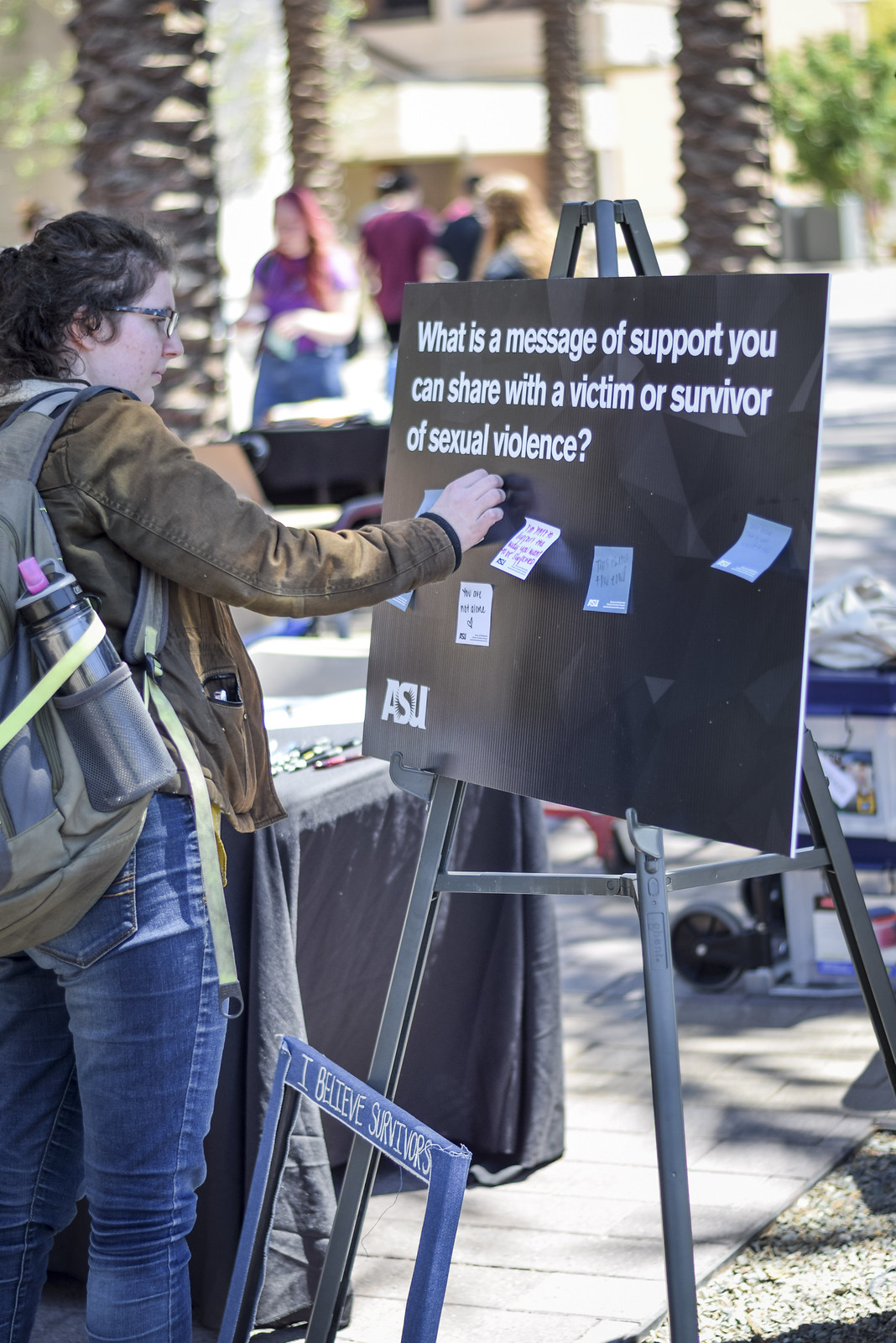In this image, a bustling outdoor scene with palm trees and people walking along the sidewalk serves as the backdrop for a small outreach event. A black message board on a metal easel takes center stage, bearing the prompt, "What is the message of support you can share with a victim or survivor of sexual violence?" The board is adorned with sticky notes of various colors, including blue and white, each containing heartfelt messages of support. At the bottom of the sign, a bold statement reads, “I believe survivors.”

To the left of the board, a woman, framed prominently in the foreground, engages with the display. She has dark brown hair, glasses, and is dressed in jeans and a brown jacket with an open pocket. Wearing a gray backpack equipped with a sport drink container, she carefully places a post-it note on the board. The scene is washed in sunlight, enhancing the vivid details of the setting and highlighting the importance of the supportive messages being shared by the participants. A table is visible behind her, suggesting additional activities or resources related to the event.